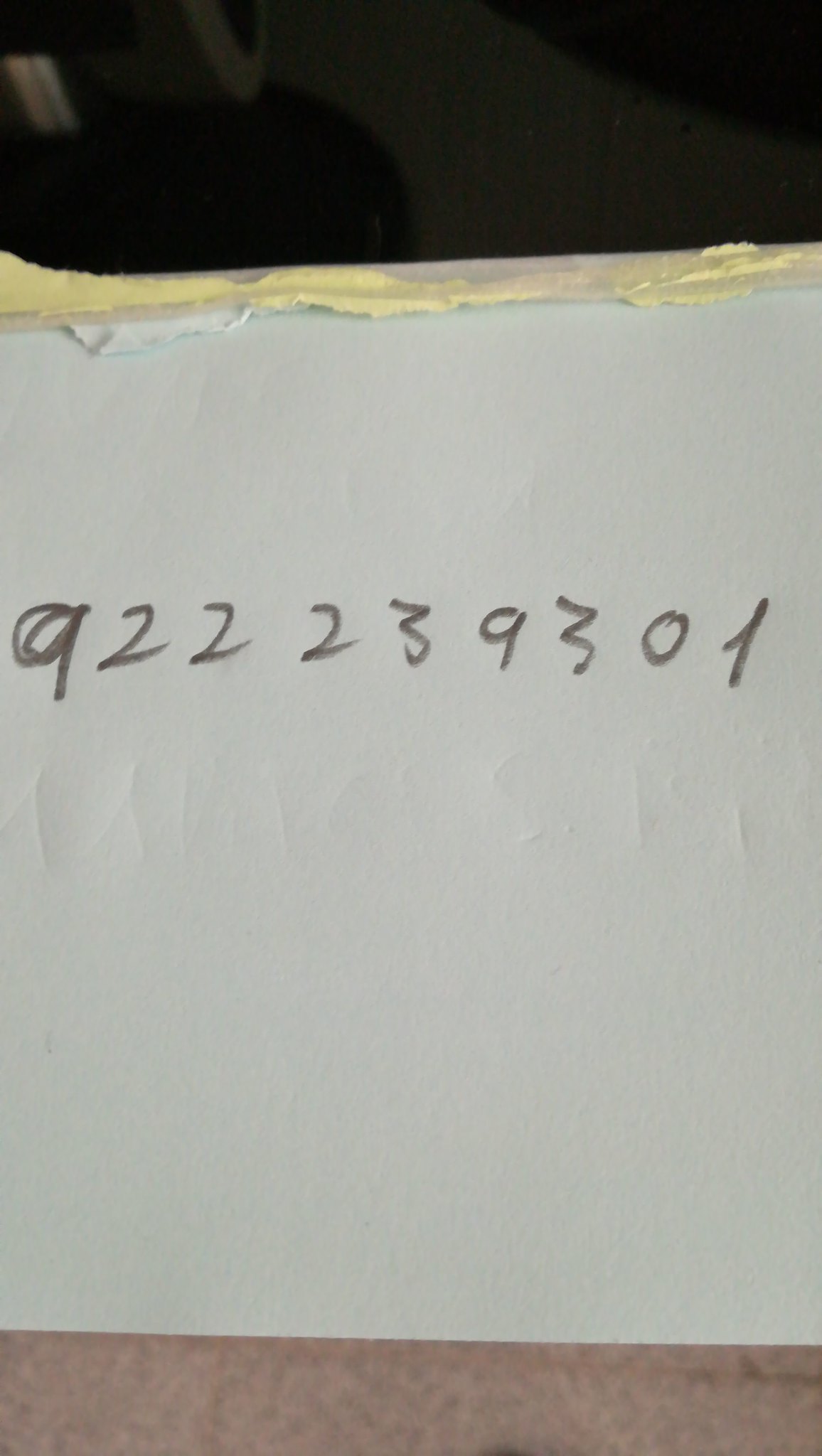This indoor photograph captures the subdued ambiance of a home setting, shrouded in darkness. Faint outlines of furniture can be discerned in the dim light at the upper portion of the image. Central to the scene is a table covered with a pink-patterned tablecloth. Atop the table lies a roughly torn sheet of thick white paper, revealing jagged edges indicative of its forcible separation from a notebook. The paper bears faint impressions of a previously written note, displaying an indecipherable sequence of numbers: 9, 2, 2, 2, 3, 9, 3, 0, 1. The barely perceptible markings suggest the remnants of an inscription once pressed upon a now-removed page.